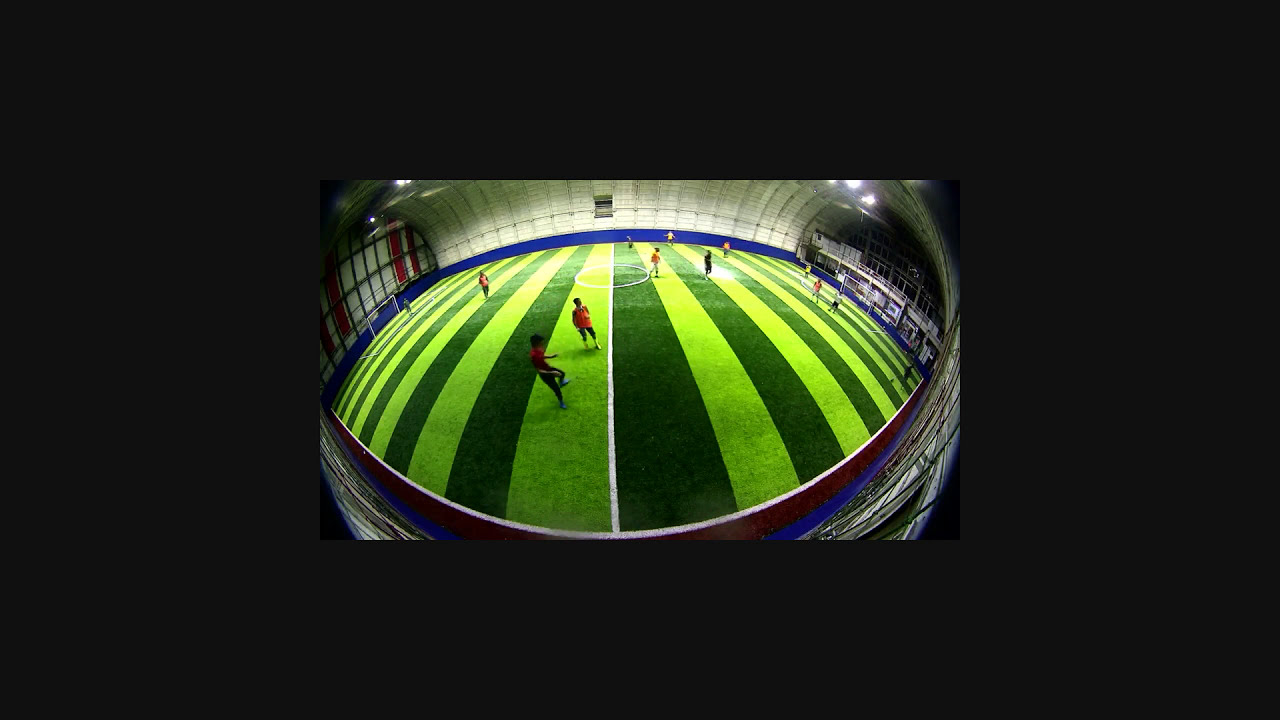The photograph captures a dynamic scene inside a spacious indoor sports stadium, likely during a soccer match. Shot through a wide-eyed lens, which gives the image curved edges, the field is distinctively marked with alternating dark and light green stripes, punctuated by a central white line and circle. Both soccer goals are visible, positioned at opposite ends of the field, but appear distant due to the lens effect. Players are actively engaged in the game, with one team dressed in red and the other in black. The stadium walls are prominent; the back wall is tall and white, while the right wall features red stripes. High stadium lights brightly illuminate the scene from above, enhancing the clarity and vividness of the image. Encasing the entire image is a thick black border. The high-angle perspective and absence of spectators suggest the possibility of a practice session rather than a live match.